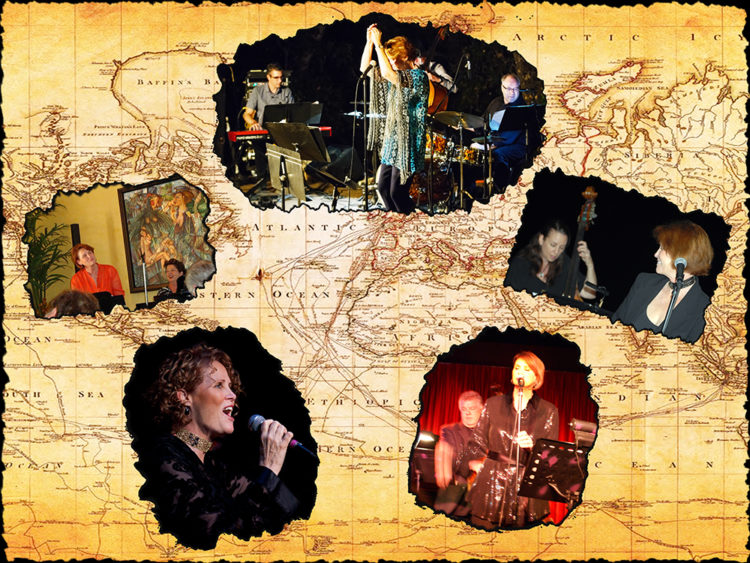The image is a visually striking collage set against a flat, two-toned map of the world in cream and yellowed brown hues, with the continents left uncolored. Superimposed on the map are five torn, jagged-edged photographs, each placed over different regions, depicting various events in the life of a white woman with ginger, sometimes curly, sometimes straight hair. 

In the photograph over the United States, the woman is at a lectern wearing a red shirt, speaking to a crowd with a painting behind her, indicating a formal event. Above Europe, she is captured mid-performance with a band, wearing a poncho-like top, clapping while singing into a microphone. On Asia, she turns her head toward another woman playing a stringed instrument, possibly a bass or cello, while she sings into a microphone, dressed in black attire. In the photograph over Africa, the woman, dressed in a belted kimono, sings into a microphone with a bandmate behind her against a red curtain backdrop. Finally, over South America, she is shown in profile, wearing a black velvet filigree jacket, singing into a microphone, her curly hair framing her face.

The five images are vibrant and collectively bring the woman's diverse experiences to life, all intricately meshed into the brown and ivory world map backdrop, creating a colorful, engaging visual narrative.